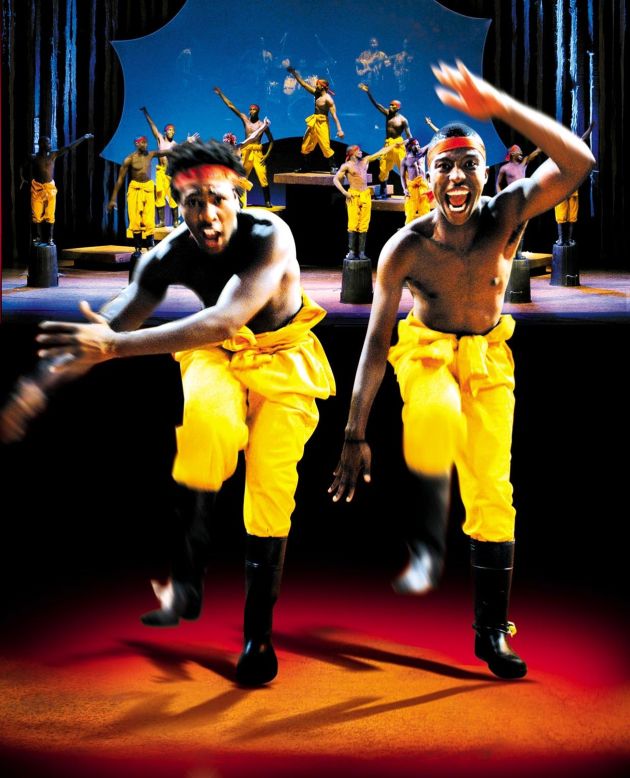The hyper-realistic, AI-generated image showcases a dynamic scene that appears to be a promotional shot for a musical or a dance troupe performance. The foreground features two shirtless black men, clad in yellow pants and black knee-high rubber boots, with gold and red headbands around their heads. The men are caught mid-dance, their blurred arms and feet vividly capturing their kinetic energy. The dark orange ground they perform on contrasts sharply with the dark blue backdrop behind them.

The stage in the background is multi-leveled, populated with numerous other dancers who mirror the attire and skin tone of the men in front. Some dancers are positioned on small buckets, while others stand on platforms, all engaged in synchronized movements. The backdrop includes a screen styled to resemble stretched animal hide, displaying an image of a group playing music. Dark blue curtains frame the stage, adding to the theatrical setting, and hinting at a performance that could be on Broadway or a similarly grand venue.